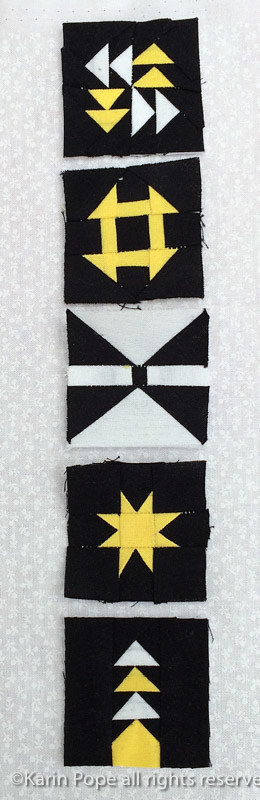This image showcases a meticulously arranged selection of five quilt blocks, all exhibiting a cohesive color palette of black, white, and yellow. The quilt blocks are displayed in a vertical column against a clean white fabric background. Each block features geometric patterns primarily composed of triangles and rectangles with an array of black, white, and yellow fabrics. Notably, the quilt pieces are individually separated and have roughly cut edges, allowing threads to extend slightly. 

The top quilt block displays an intricate design of eight triangles radiating outward with alternating white and yellow colors. The second block is distinguished by its solid yellow shapes. The third block, featuring a predominance of white against black, contains a symmetrical arrangement of white triangles and strips. The fourth block has a striking design with a central yellow star composed of triangles within a black fabric backdrop. The final block is set off by alternating white and yellow triangles. 

At the bottom of the image, overlay text in white reads "© Karen Pope All Rights Reserved," asserting the image's copyright. The artistry and precise geometry of each quilt block exemplify a detailed and harmonious composition, making this a striking representation of quilt pattern designs.